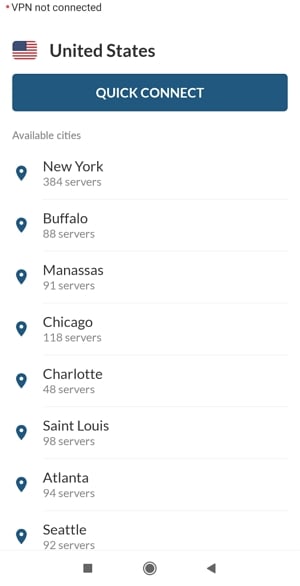The image displays a VPN (Virtual Private Network) website interface. At the top, there is a prominent "Quick Connect" button. The header indicates "VPN Not Connected" and provides a selection of available cities displayed in gray. 

New York, which is presented with 384 servers, stands out with its name in bold and black. Each city's server count is in gray text with a blue pin icon to the left of the city name. Below New York, the city names and the number of servers are as follows: Buffalo with 88 servers, Manassas with 91 servers, Chicago with 118 servers, Charlotte with 48 servers, St. Louis with 98 servers, Atlanta with 94 servers, and Seattle with 92 servers. There is a dividing line between each city's details.

At the bottom of the interface, there is an icon section that includes a double circle, a solid circle with an outlined circle around it, and a back button to the left. The map of the United States is depicted in traditional red, white, and blue colors, with a blue square and white stars. The background of the interface is white.